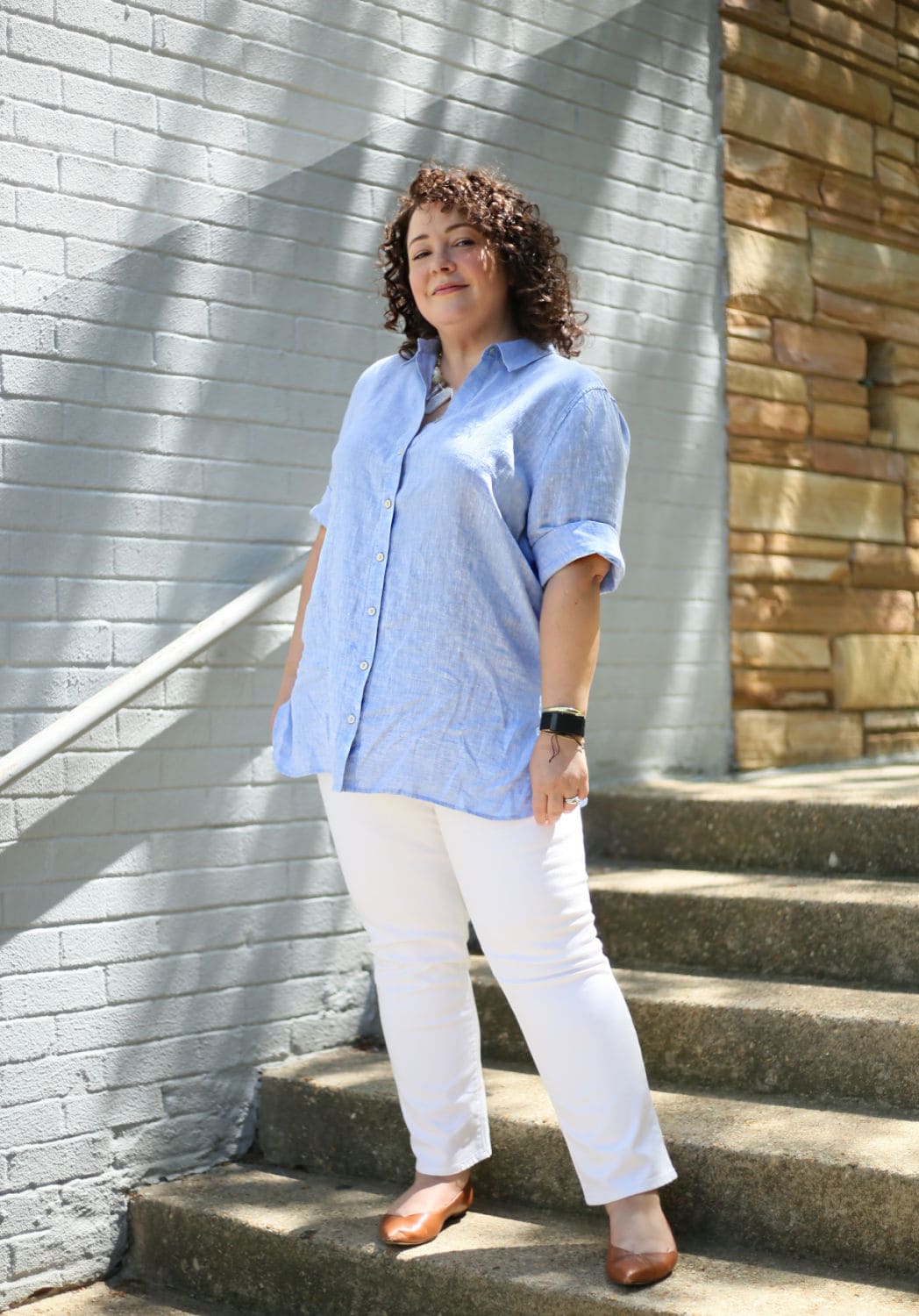In the image, a plus-size woman stands confidently on a set of gray cement stairs in a courtyard. She is positioned on the fourth step from the bottom, leaning against a section of the backdrop that includes a white brick wall on her left, transitioning into a mix of orange and yellow bricks above. The right-hand side features a distinctive light blue railing with an adjacent light blue wall, which shifts into a brown stone structure higher up.

The woman, estimated to be in her 30s to 40s, sports curly black hair and a smug expression. She is dressed in a light blue, men's collared button-up shirt, which is untucked and loose around her midriff, with the sleeves rolled up to her elbows. She also wears wide-legged white slacks and pointed brown flats. Accessories include a black watch on her left wrist and a ring on one of her fingers. Despite the contrasting background, her poised stance and detailed outfit draw the viewer's attention.